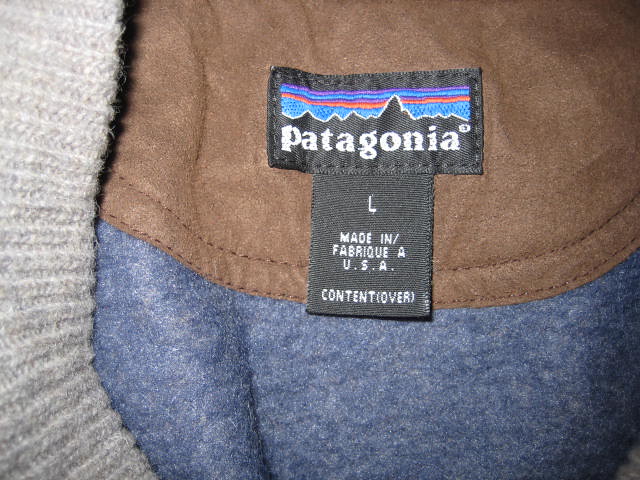A close-up photograph captures the intricacies of a clothing tag affixed to a piece of knitwear. The garment features a textured gray knit section on one side, transitioning into a navy fabric, and then into a chocolate brown section. The focal point is a tag sewn onto the chocolate brown part of the material. This tag prominently displays the brand name "Patagonia" in white font, set against a vivid backdrop depicting a black mountain range outlined in white with a sky gradient in shades of blue, red, and purple. Directly beneath, a smaller black tag is sewn, bearing the text "L, Made in USA" in white, along with instructions to flip the tag for additional information. The high-quality image also captures the camera flash reflecting on parts of the fabric, emphasizing the detailed stitching along the top of the Patagonia tag.